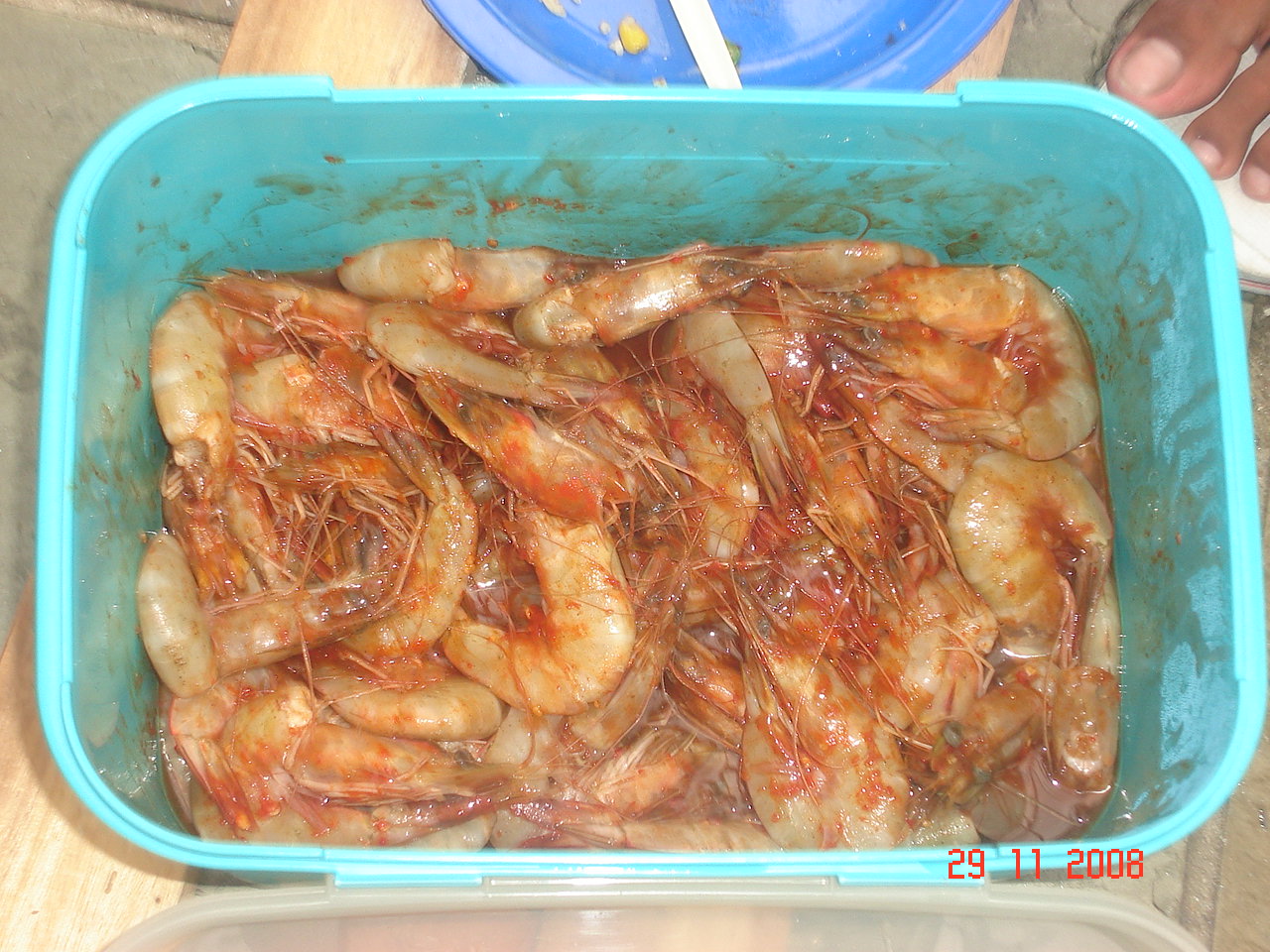The image, taken with a digital camera and timestamped November 29, 2008, depicts a scene centered around a rectangular, turquoise plastic storage container, approximately 10-gallons in size. The tote, possibly made by brands such as Totes or Sterilite, is filled with shrimp that still have their heads and tails intact, marinating in a wet, red chili sauce. The container features an attached lid. In the lower part of the image, the container is placed on a wooden platform, with some of the gray ground visible in the background. To the top right, the foot of a person with black skin, possibly wearing flip-flops, is partially visible, showing the big toe and two smaller toes. Next to the person’s foot, there is a white object, possibly a bucket, which may contain a piece of corn. The image captures a snapshot of a moment focused on food preparation or marination against a rustic backdrop.